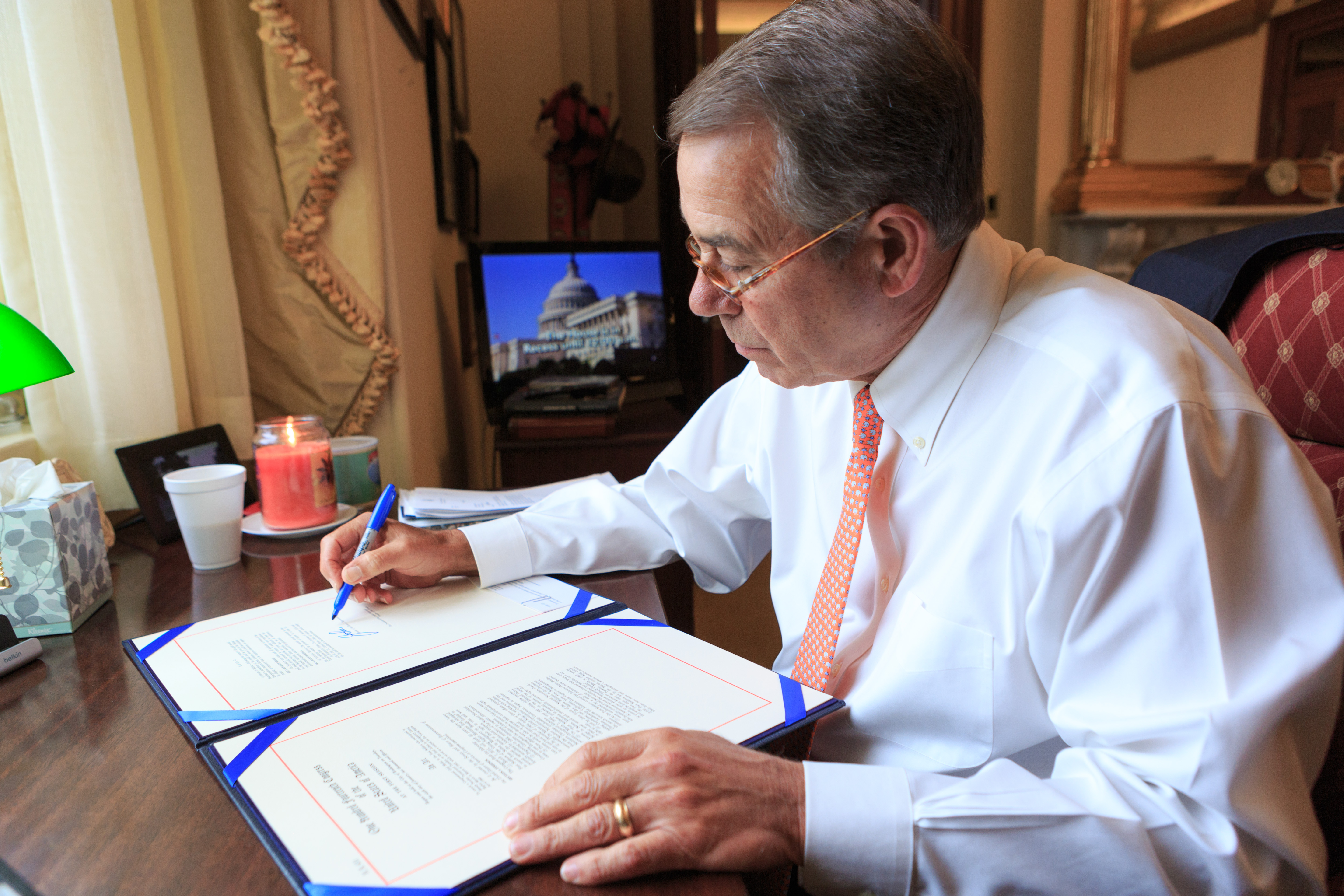In this detailed photograph, an elderly man, possibly a politician, is seated at a desk and appears to be engaged in a formal activity, such as signing important documents. The man is well-dressed, wearing a meticulously ironed, long-sleeved white shirt paired with a distinctive thin orange tie. He has short gray hair and glasses, and a wedding ring is visible on his left hand.

On the desk in front of him lies an open booklet resembling a professional or legal document, adorned with blue ribbons, reminiscent of a graduation certificate. He is signing this document with a blue felt pen, possibly a Sharpie marker. In the background, a TV or computer screen displays an image of the White House, reinforcing the impression that this man works in a significant governmental or political capacity.

Additional items on the desk include a half-drunk Styrofoam cup of coffee, a photograph in a frame, a box of tissues, and a lit red or pink candle. A green desk lamp provides ambient light, while a turquoise canister and other papers are scattered about. The man is seated on a red chair with his blue suit jacket draped over the back, adding a touch of personal comfort to the formal setting.